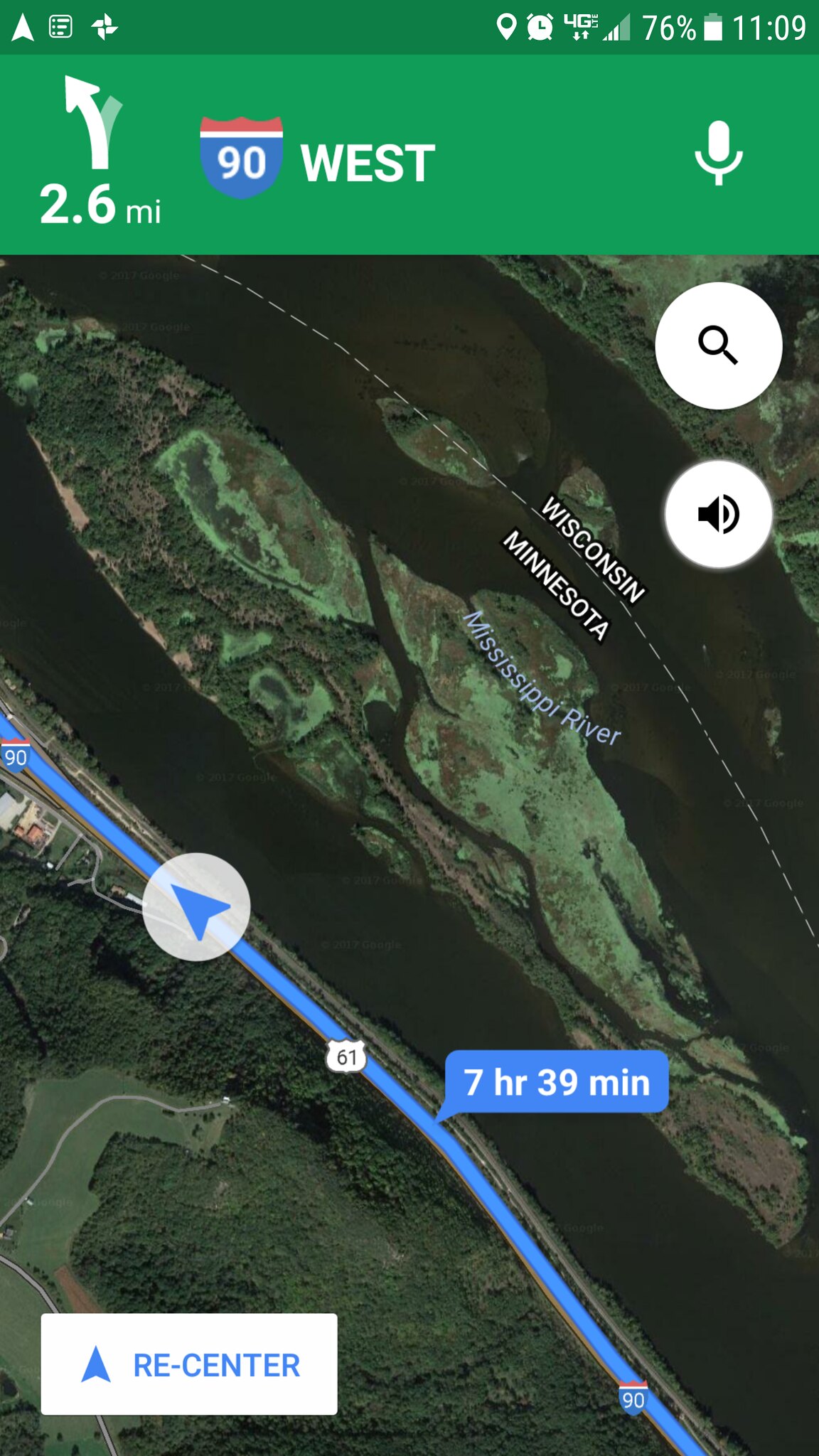A cell phone screenshot from a mapping application, likely taken on an Android device, shows a topographical map with satellite imagery, depicting the state line between Wisconsin and Minnesota, separated by the Mississippi River with its delta islands. The river, running vertically toward the center of the image, has "Minnesota" labeled to its left and "Wisconsin" to its right. At the top of the screen, a dark green banner displays typical phone status icons including the battery at 76%, the time at 11:09, and the 4G signal. A lighter green strip directly below this contains a red, white, and blue interstate sign marking "90 West" accompanied by a left-curving white arrow indicating 2.6 miles to go. To the right, there's a white microphone icon for voice commands, and further right, search and speaker icons. The map features a blue route line extending from the lower right to the center left, marked as Interstate 90 and Route 61. A white circle with a blue directional arrow indicates the current path, with a time estimate of 7 hours and 39 minutes displayed next to it. In the bottom-left corner of the screen, a "Re-center" button in a white rectangle with blue text is visible.